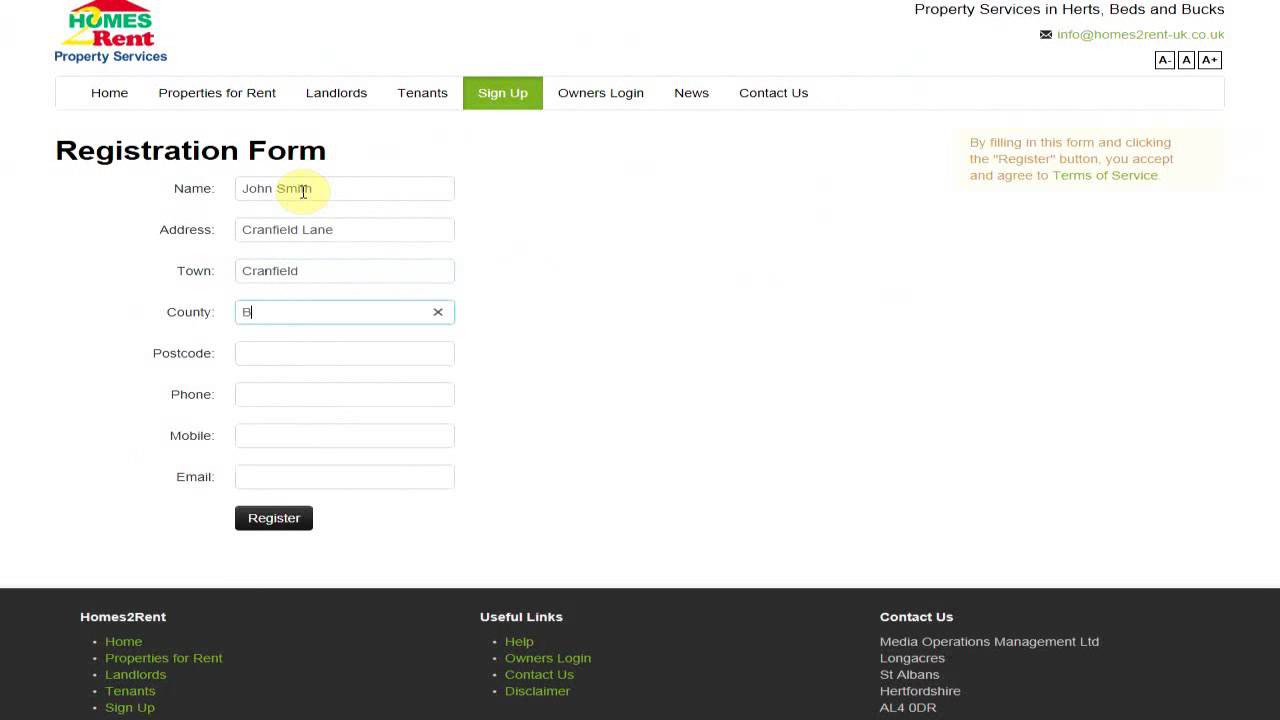The screenshot captures a website interface. In the top left corner, a logo is displayed alongside navigation options labeled "Homes," "Rent," and "Property Service." On the right side, there is text reading "Property Services in Hertz, Bits, and Bucks." The website appears to be for a UK-based service, with contact information listed as "info@homestorent.uk.co."

Below the top navigation, a secondary menu features tabs for "Home," "Properties to Rent," "Landlords," "Tenants," "Sign Up," "Owners Login," "News," and "Contact Us." The screenshot specifically focuses on the "Sign Up" tab, which stands out with its green background in contrast to the otherwise white background of the page.

Below the "Sign Up" tab, there is a registration form to be filled out. The form includes fields for "Name" (filled in as John Smith), "Address" (Cranfield Lane), "Town" (Cranfield), and "County" (currently being filled out). Fields for "Postcode," "Phone," "Mobile," and "Email" remain empty. At the bottom of the form, a black "Register" button is prominently displayed.

The bottom section of the screenshot also features a black background with links typically found in the footer, including "Contact Us" and other relevant information.